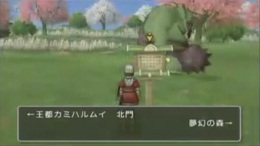This image is a detailed in-game screenshot set in a colorful landscape. Dominating the scene is lush green grass which covers a significant portion of the image. In the foreground, facing away from us, there's an in-game character clad in a reddish jacket or cloak along with a white hat. This character is interacting with another figure directly in front of them. To the right of this main interaction, there's a small figure in a brown outfit and an additional creature partially obscured, possibly behind a shelf or a desk.

In the background, vibrant hues adorn the environment; trees with light pink cherry blossom-esque leaves, white foliage, and some with green leaves provide a diverse palette. The sky transitions from a yellow tint to blue, predominantly on the left and upper left parts of the image. Peaks of sharp hills are visible across the upper section of the scene, from left to right, adding depth to the landscape.

A key feature on the bottom center of the screen is a black transparent chat dialog box, bordered in white, containing text in Japanese characters, adding to the immersive in-game experience.